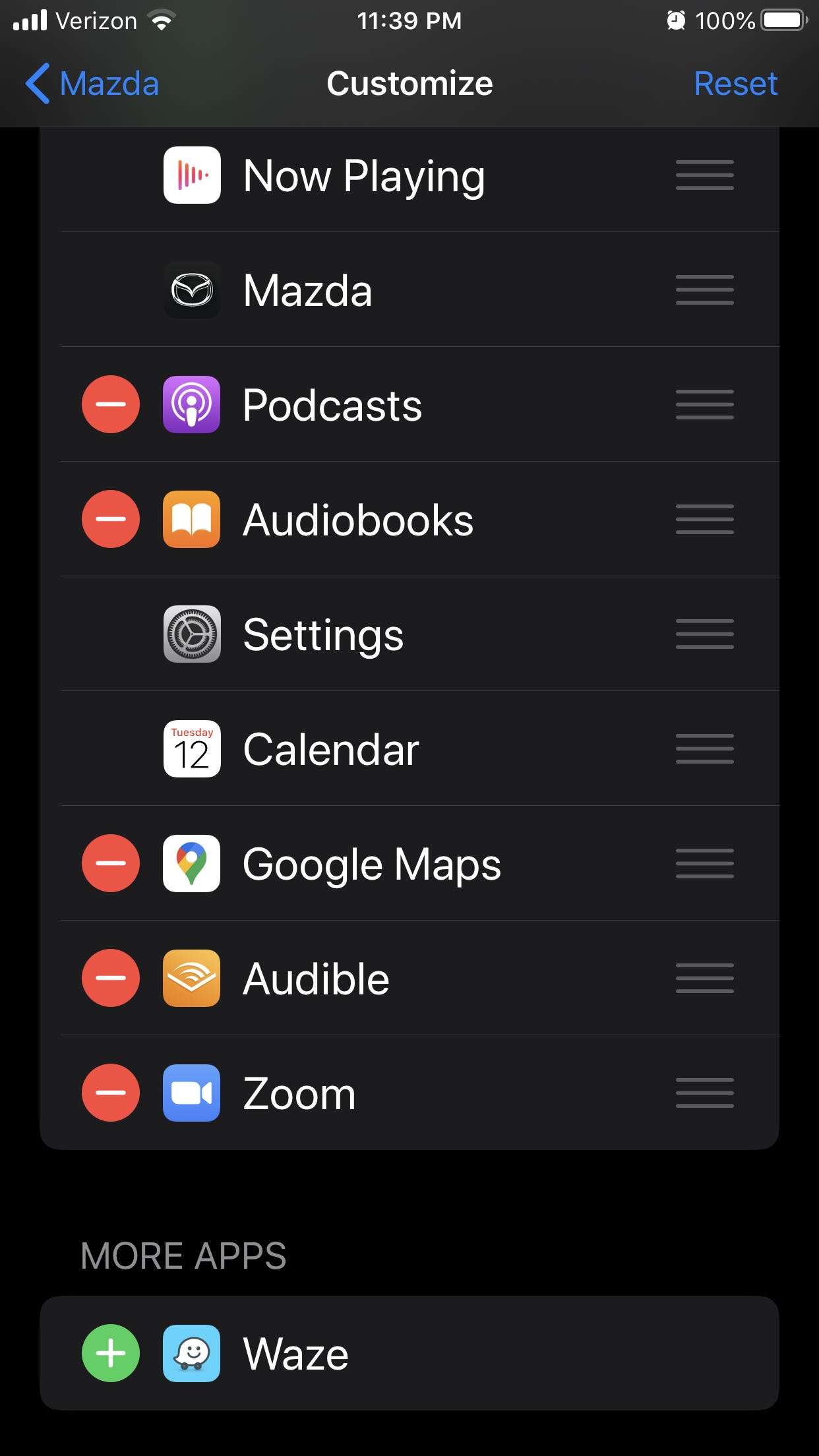Screenshot of a phone interface displaying various customization options. 

**Status Bar:**
- **Top Left:** Signal strength indicator with four bars of increasing height, followed by the text "Verizon" in white.
- **Next:** WiFi signal indicator represented by a circle with two lines above it.
- **Center:** The current time displayed as "11:39 PM."
- **Top Right:** An alarm clock icon, battery status showing "100%" with a full battery icon.

**Main Customization Options:**
- **Left Section:**
  - A blue outlined arrow pointing left with the text "Mazda" in blue.
  - A white text "Customize" centered.
  - "Reset" in blue text to the far right.

**App Shortcuts:**
- **Audio & Navigation:**
  - **Now Playing:** White box with a left-pointing arrow made of several small red lines and "Now Playing" in white text.
  - **Mazda:** Black box with a white Mazda logo, "Mazda" in white text.
  - **Podcasts:** Red circle with white line next to a purple box with a white symbol of an eye intersecting two circles, and "Podcasts" in white text.
  - **Audiobooks:** Red circle with white line next to a yellow box with a white book icon, and "Audiobooks" in white text.
  - **Settings:** Grey box with a black gear icon, and "Settings" in white text.
  - **Calendar:** White icon with a black number 12, "Calendar" in white text.
  - **Google Maps:** Red circle with white line next to a white box with a multicolored map pin made from the Google logo, and "Google Maps" in white text.
  - **Audible:** Red circle with white line next to a yellow box with an open book icon and three white lines between the pages, "Audible" in white text.
  - **Zoom:** Red circle with white line next to a blue icon with a white camera, "Zoom" in white text.

**Additional Options:**
- **More Apps:** White text "More Apps" followed by a black box with a green circle and a white plus symbol inside.
- **Waze:** Blue box with a white symbol inside followed by "Waze" in white text.